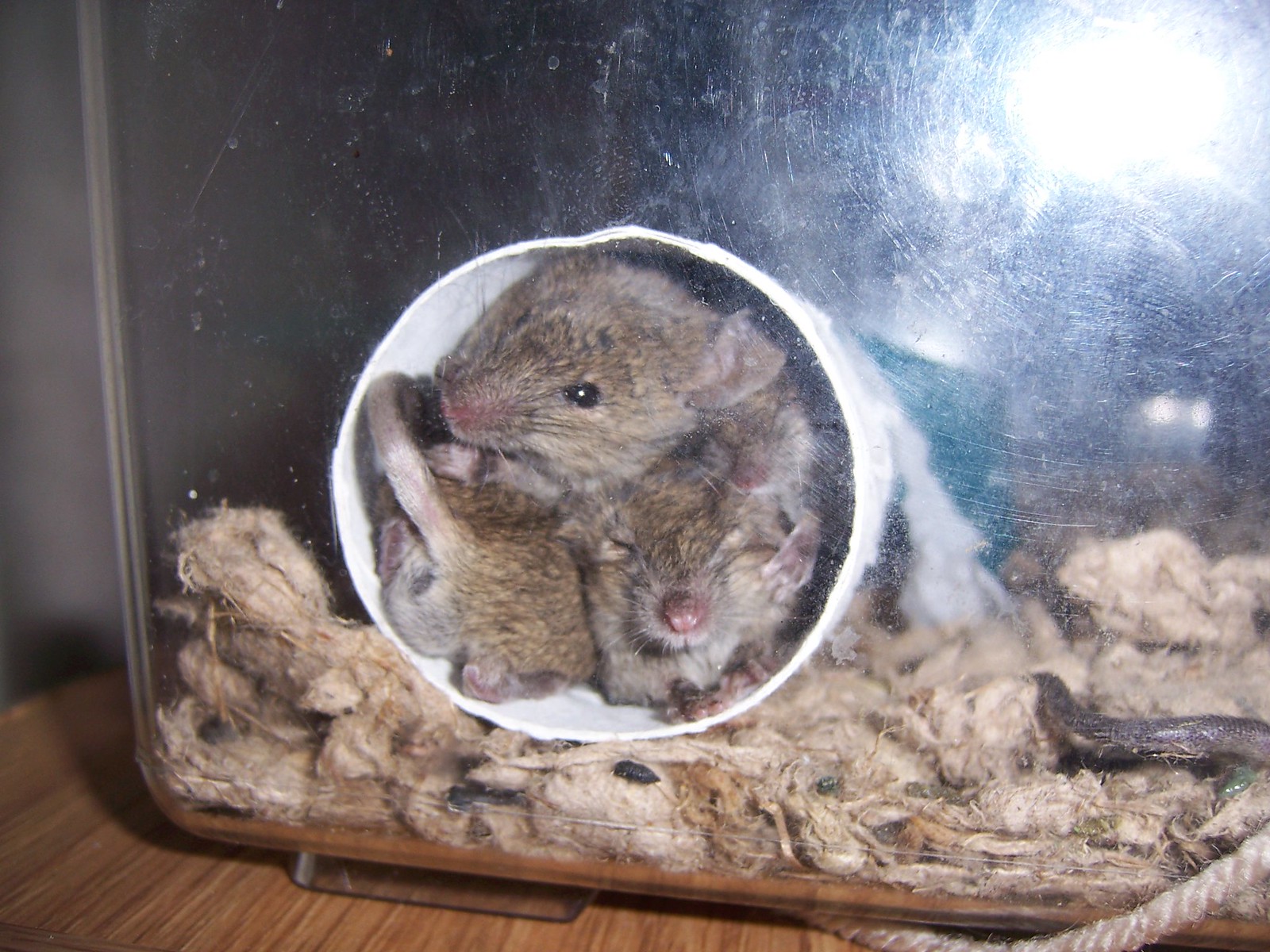In this detailed image, a glass-encased habitat sits on a brown wood-grain table, setting the stage for a scene featuring three small animals. These creatures, identified as traditional hamsters with brown, gray, and tan fur, have crammed themselves inside a round, white cardboard tube. Their pink noses stick out, with two of the hamsters facing outward and the third one's tail protruding. One hamster appears to have its eyes shut, possibly asleep, while another looks directly at the camera. Below the tube, brownish fabric and what appears to be a rope are visible, adding texture to their cozy space. The background includes wood chips, enhancing the naturalistic feel of the cage. A flash from the camera reflects off the glass, particularly in the upper right quadrant, slightly obscuring part of the image.